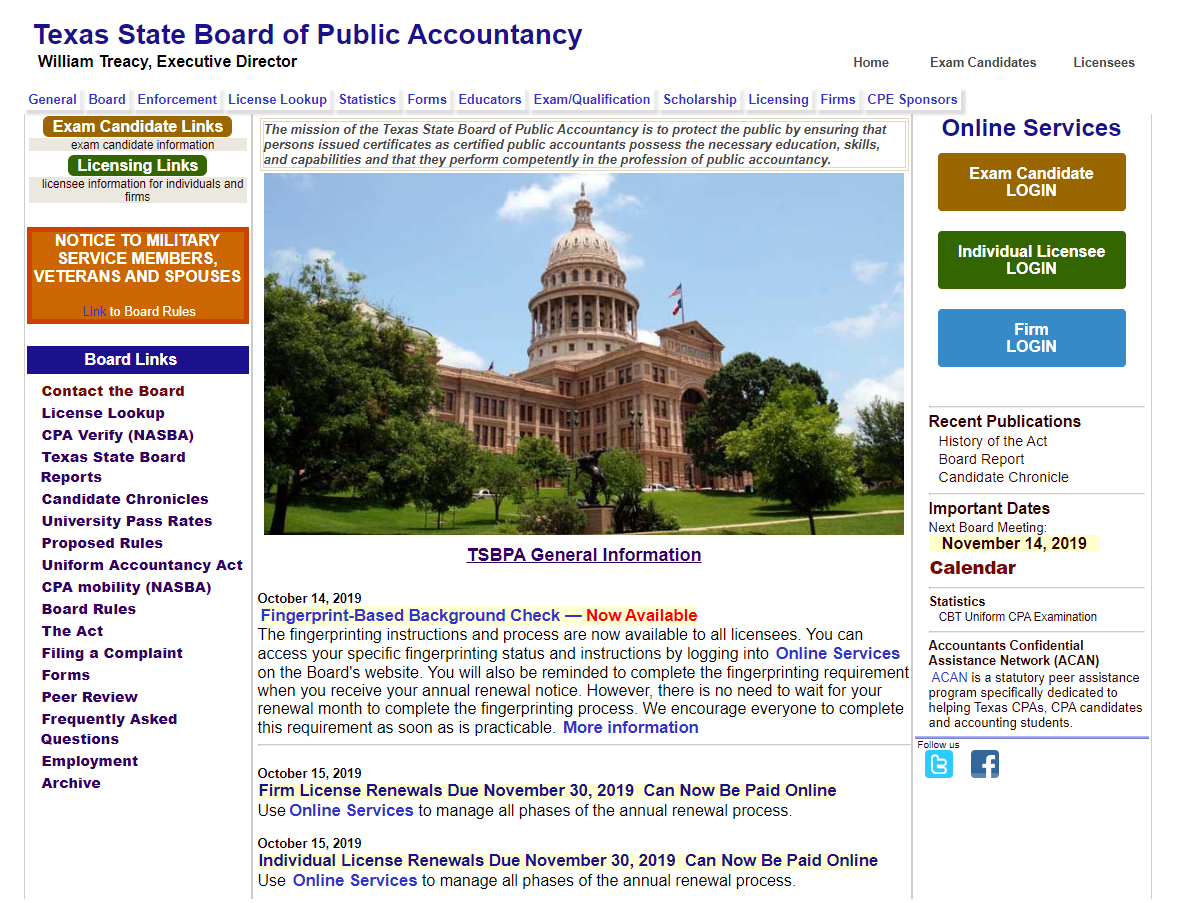The caption describes the Texas State Board of Public Accountancy's official website. At the center is an image of the Texas Capitol building, its classic architecture highlighted against a clear, daylight sky. The building is framed by a lush green lawn and topped with the Texas and United States flags. A statue is visible at the base of the building, adding to the historic ambiance.

The website is designed to serve various stakeholders within the public accountancy profession. To the left of the central image, there are links for exam candidates and licensing information, with a notable orange background section highlighting special notices for military service members and their spouses. Key links listed include contact information for the board, a license lookup feature, CPA verification, board reports, university pass rates, information on CPA mobility, board rules, the governing act, procedures for filing complaints, forms, FAQs, peer review details, employment opportunities, and archives.

The page is dated around October 14, 2019, marked by a notice for new fingerprint-based checks available to licensees, with instructions accessible through the board’s online services. On the right side of the page, login sections cater to exam candidates, individual licensees, and firms. There are also announcements for recent publications and upcoming important dates, including a board meeting scheduled for November 14, 2019. The top of the page features navigation buttons for home and licensees.